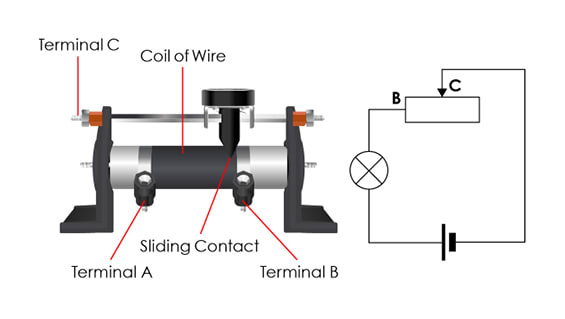The image illustrates a detailed diagram of a small piece of electrical machinery featuring a central cylindrical metal component housed between two brackets. This cylinder includes a coil of wire and is flanked by three labeled terminals: Terminal A at the bottom, Terminal B also at the bottom but in a separate black housing with a silver contact point, and Terminal C positioned at the top left. A sliding contact, described as a black piece with a silver element, is affixed at the top.

On the left-hand side of the image lies the physical depiction of the machinery, while the right-hand side presents a simplified electrical drawing that outlines its functional flow. This schematic includes a rectangle formed by black lines, with Terminal B and Terminal C marked at the top. An arrow from C points into the rectangle, suggesting an input or flow direction, and the broader black lines at the bottom signify the termination of the circuit. Additional details on the schematic include a Phillips head screw in the upper left corner, providing context for assembly or connection points. The combined visual elements imply this is an electrical device designed to facilitate or control current through its sliding contact and terminals.